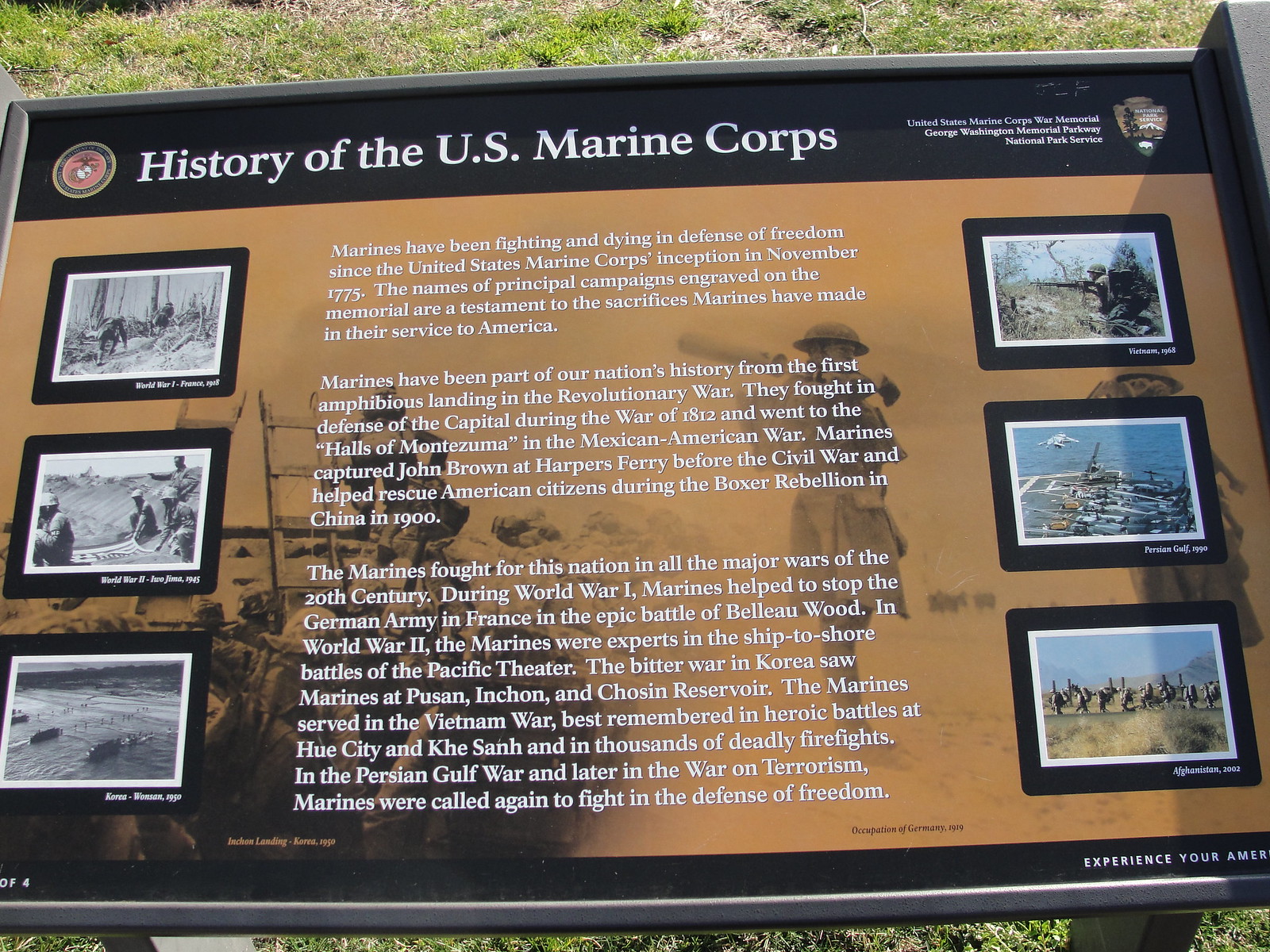The image depicts a plaque titled "History of the U.S. Marine Corps," mounted on a metal stand anchored in a grassland. The plaque features six photographs: three black and white images on the left and three colored images on the right. The top two black and white photos depict Marines in action, while the bottom image shows ships at sea. Similarly, the color photos on the right also display Marines and maritime scenes. Centered on the plaque are three paragraphs printed in white text. The text begins, "Marines have been fighting and dying in defense of freedom since the United States Marine Corps inception in November 1775." It details the Marines' involvement in significant campaigns, their sacrifices, and their enduring presence in American history, from the Revolutionary War to modern times. The plaque is framed by Marine Corps symbols, underscoring its commemorative purpose.